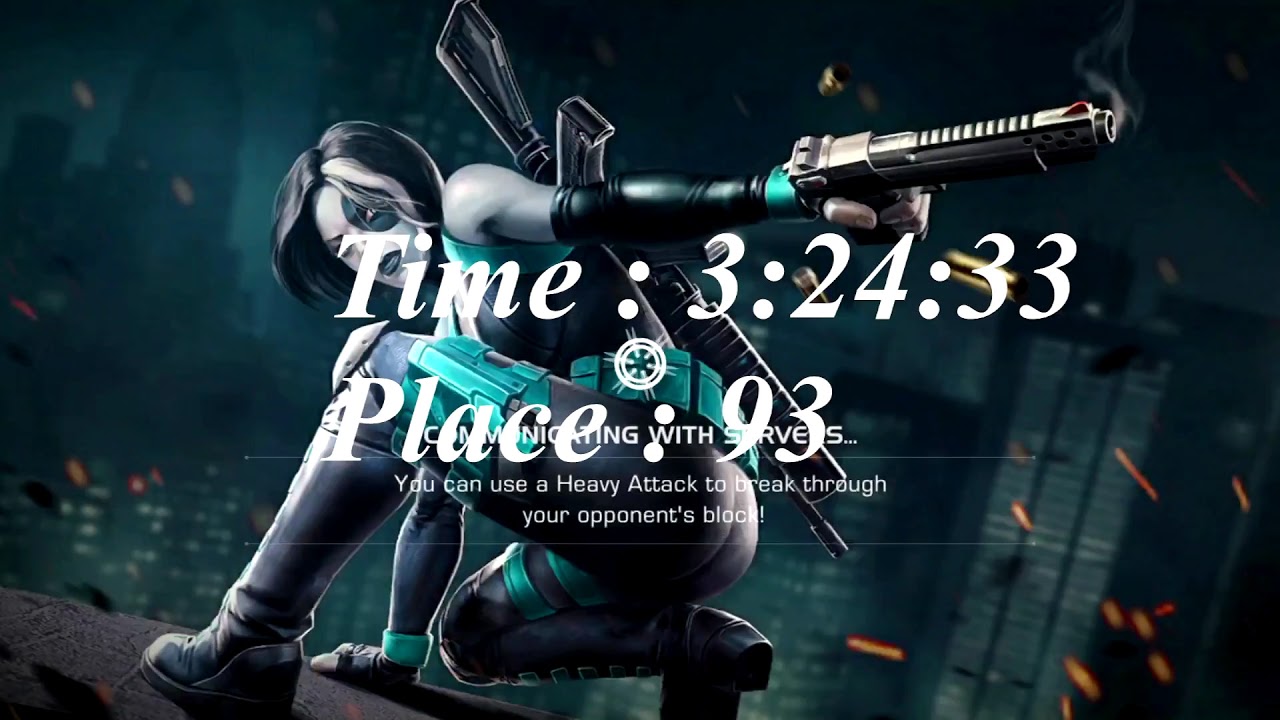The image is a detailed screenshot from a video game, presenting a digitized, cartoon-like depiction of a female character against a dark green, blurred cityscape backdrop with indistinct skyscrapers. The scene is set at night on a rooftop, marked by grayish silver skin and striking short black hair with a prominent white streak. The character, a superhero-like figure, wears a form-fitting black leather bodysuit with lighter green accents and green makeup, including a patch around one eye and green lipstick. She is crouched, propped on one knee with the other bent, holding a golden-colored gun aimed towards the upper right corner, where bullets and orange sparks are visible. Additional weapons, including a rifle and a sword, are strapped to her back. Accompanying the visual are white text overlays displaying "Time: 3:24:33, Place: 93," and a note reading, "You can use a heavy attack to break through your opponent's block," indicating possible in-game hints or instructions.